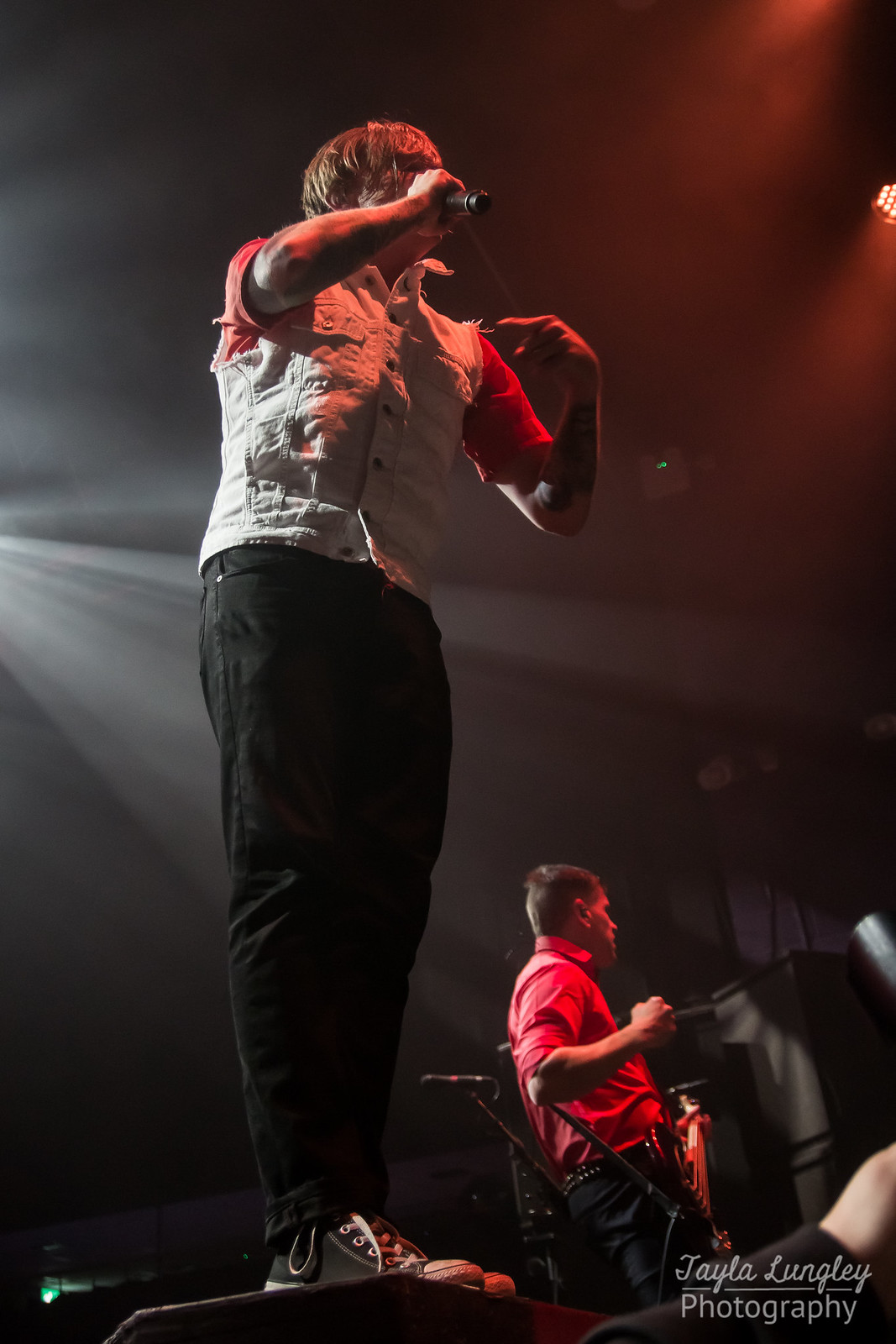This photograph, credited to Taylor Lungley Photography, captures the vibrant energy of a concert. Dominating the foreground is a singer with short brown hair, dressed in a white shirt paired with black pants and black sneakers, gripping a microphone in his right hand. The singer stands confidently on stage, illuminated by various stage lights including a prominent white spotlight and additional red and white floor lights. To his left, there's a guitarist clad in a red shirt—described alternately as short or long-sleeved with rolled-up sleeves and potentially a vest-like alteration—black pants, and black shoes. This musician is bathed in a ceiling light that highlights his presence. The sleek black background frames the performers perfectly, and at the bottom right corner of the image, an audience member's arm is also visible. The vivid lighting setup enhances the dynamic atmosphere of this musical show.